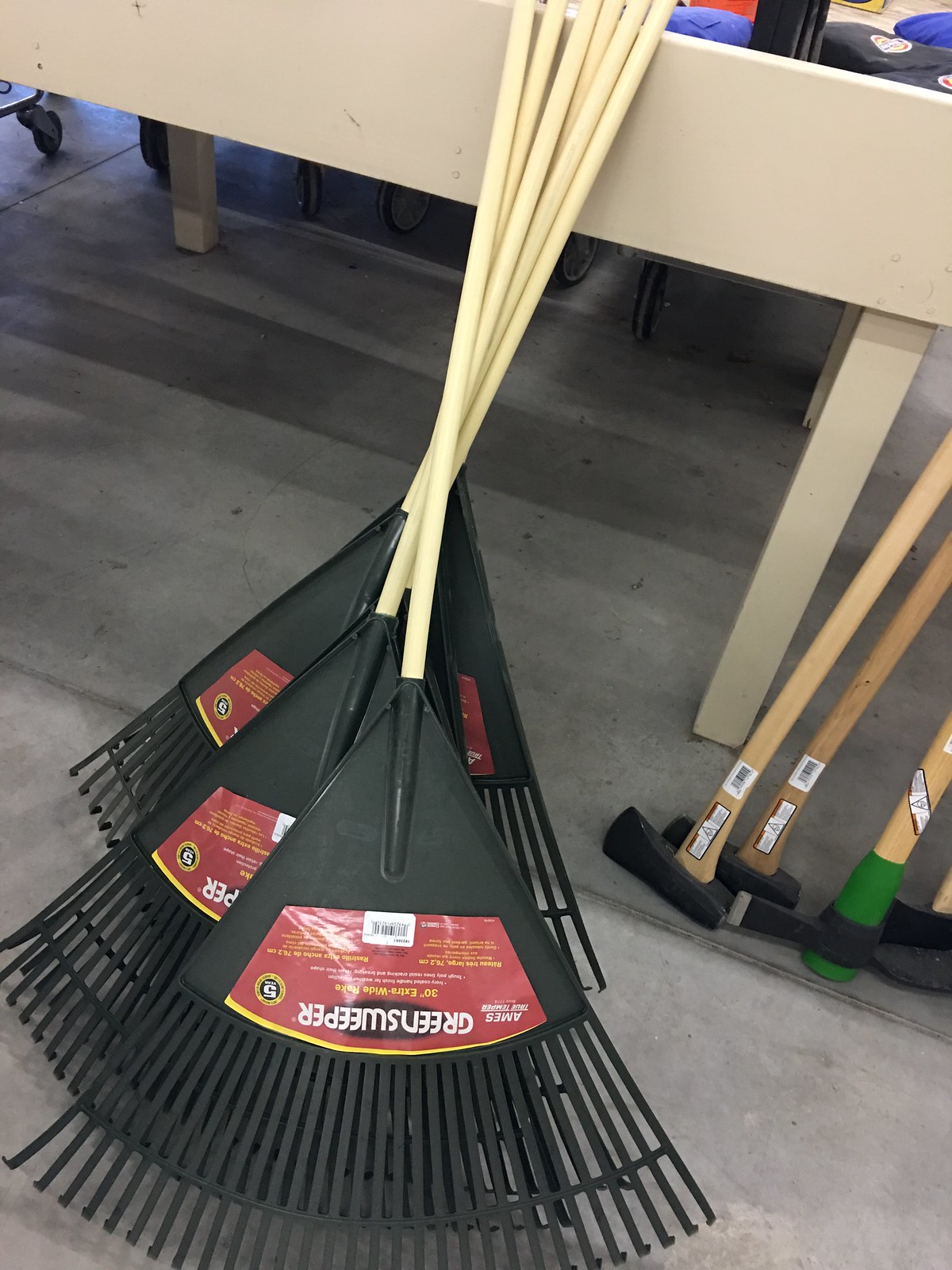In this color photograph taken inside a hardware store, we see a collection of black-headed leaf brooms and rakes leaning against a simple, cream-colored display table constructed with two-by-fours for legs. Each rake and broom displays a label that reads "Green Sweeper" in white text on dark red and yellow labels. The handles of both the brooms and rakes are thin cylinders in a light, yellowish cream color. The bristles of the brooms are made of black plastic, while the rakes feature black prongs. The table has some indistinct items on top at the top right corner. At the bottom right of the image, leaning against the table, there are several tools with wooden handles, including axes and a pickaxe. The blades of the tools are black, with the head of the pickaxe displaying a hint of green. The entire scene is set on a gray concrete floor.